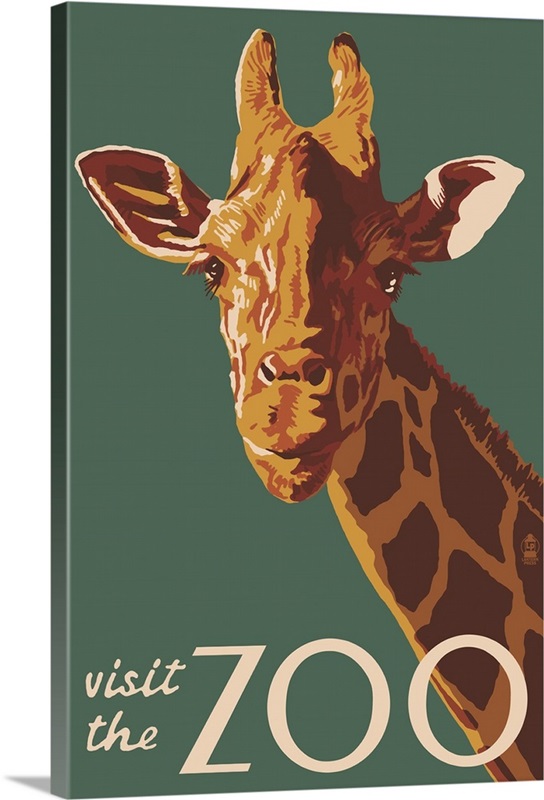This image features a stylized depiction of a giraffe on what appears to be either a book cover or a stretched canvas. The background is a deep, medium green with a possible 3D modeling texture. The giraffe, portrayed in bright orange-yellow and burnt orange shades, gazes directly at the viewer, its head and upper neck emerging from the lower right-hand side and extending towards the middle of the composition. The giraffe's distinctive spots and shading add to the detailed yet stylized aesthetic of the image. At the bottom, in a beige area, the phrase "Visit the Zoo" is inscribed. "Visit the" appears in cursive, stacked in the lower left corner, while "Zoo" is printed in a larger font, stretching from the center to the right. The canvas itself is angled slightly to the right, enhancing the dynamic presentation of the giraffe artwork.